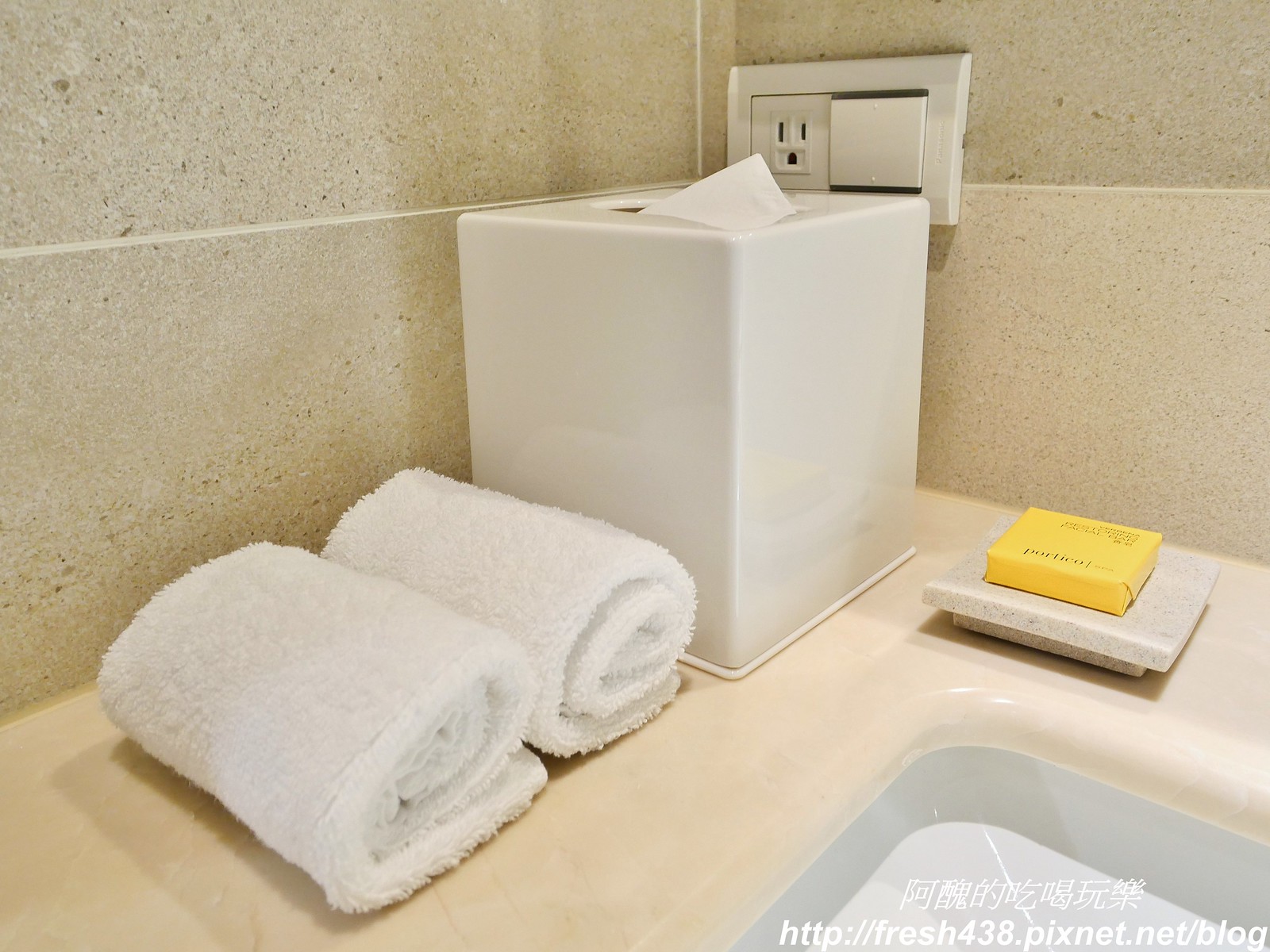This stock photo captures a close-up of a corner bathroom, focusing on the detailed textures and arrangement within. The walls are adorned with large beige granite tiles separated by white grout lines, adding a distinct and clean aesthetic to the space. Located in the corner of the image is a single electrical outlet, and adjacent to it, on the right, is a sizable square switch for controlling the overhead light.

In the foreground, a vertical white canister designed to hold tissues stands prominently, its material indeterminate but suggesting a sleek finish. Flanking the tissue canister are two neatly rolled, pristine white washcloths, emphasizing the cleanliness and orderliness of the setting. Additionally, a bar of soap rests on an elevated granite slab, providing a subtle touch of elegance and functionality.

The overall arrangement suggests this area is part of a sink setup rather than a bathtub, given the proximity to the electrical outlet. Notably, etched into the scene is a web address—http://fresh438.pixnet.net.blog—hinting at the image's association with an Asian blog, possibly offering insights into modern bathroom designs.